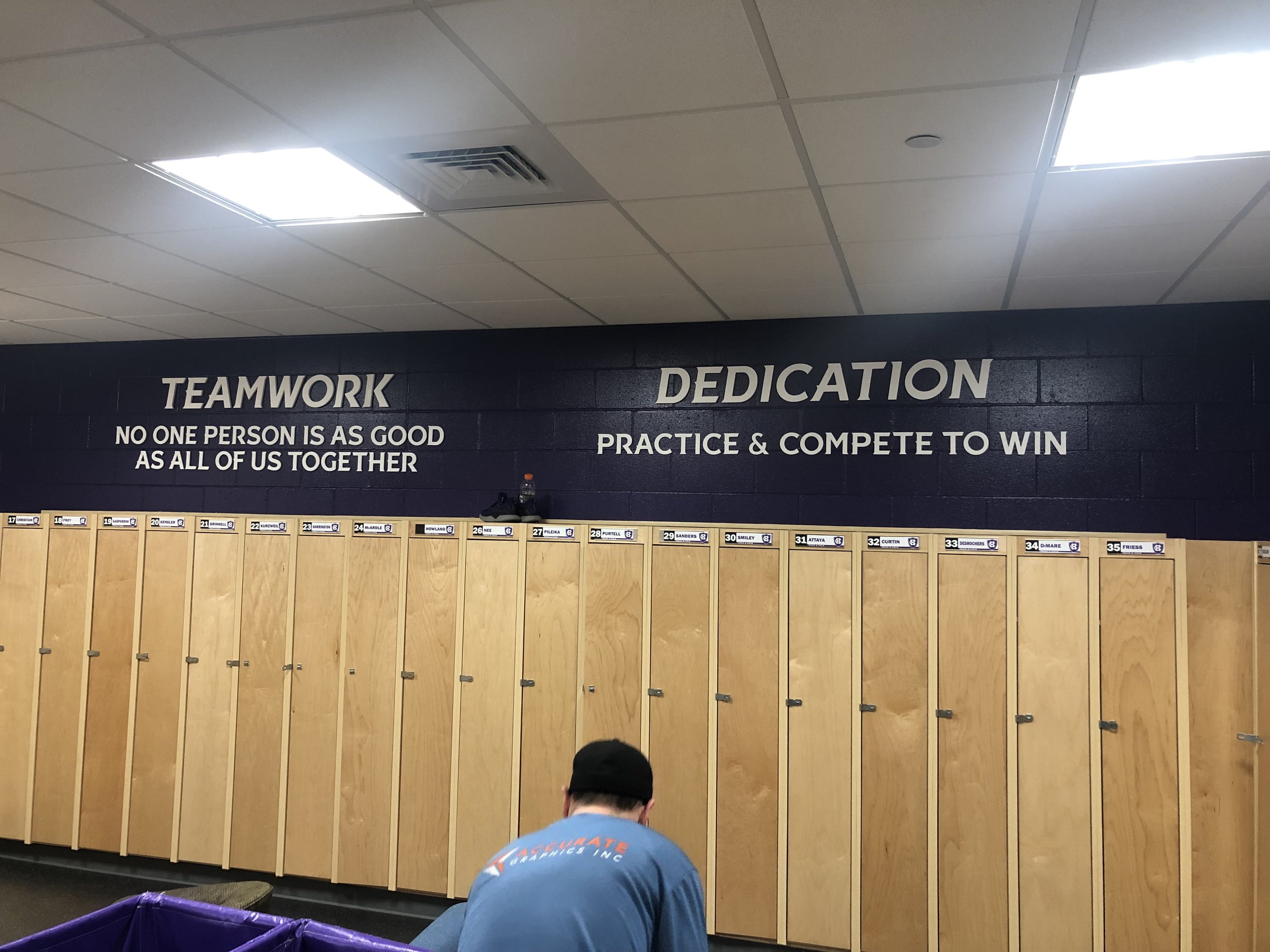A detailed indoor scene of a locker room with white tile ceilings and fluorescent lights, featuring dark blue cinder block walls. Prominently displayed on the left side of the wall, large white capital letters read "TEAMWORK," with the phrase "No one person is as good as all of us together" directly below it. On the right side, at the top, "DEDICATION" is written in similar white capital letters, with "PRACTICE" and "COMPETE TO WIN" underneath. The ceiling has tile for soundproofing and includes two lights and a fan opening. Beneath these motivational messages, there are rows of beige wooden lockers, each numbered and featuring names. Visible numbers include at least 17 through 35, with some skips in the sequence. A Caucasian man with short dark hair, wearing a light blue t-shirt with unreadable text on the back, and a black cap, is seen bent over, possibly adjusting his shoes or changing clothes. The floor appears to be black, enhancing the clarity of the scene.